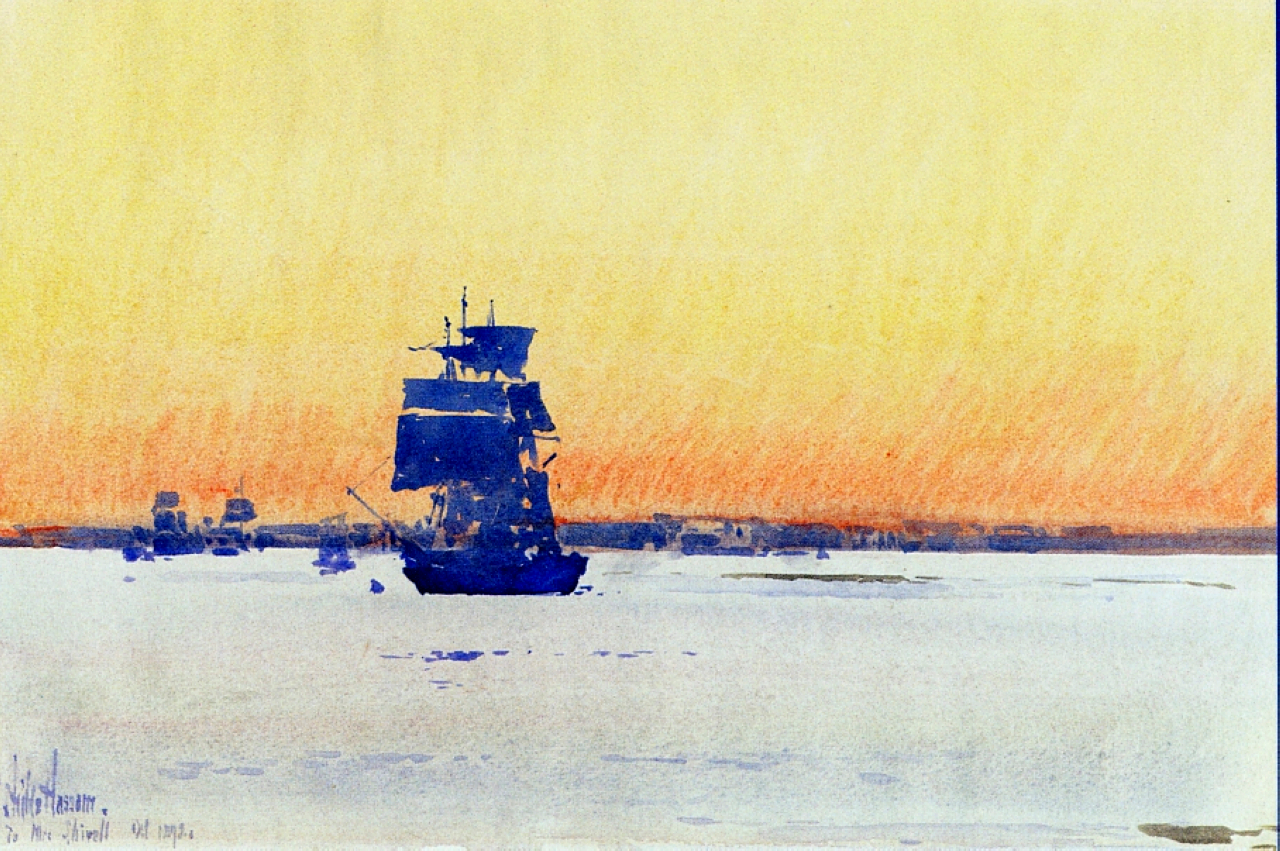This detailed painting depicts a stylized nautical scene with a serene yet vibrant atmosphere. Dominating the composition is a large boat with four to five sails, rendered in dark, indigo hues that create the impression of a shadowy silhouette against the backdrop. The boat rests on a body of water that radiates primarily white tones with subtle hints of blue. Smaller boats are scattered in the background, appearing as rudimentary shapes, adding depth to the scene. In the bottom left corner, a few weeds protrude, possibly indicating the proximity to land, though there is ambiguity if land is in the far distance or not. The horizon is imbued with a rich deep orange, seamlessly fading into a lighter yellow as it rises, evoking a sense of a daybreak or sunset. This gradient sky further enhances the painting’s dreamlike, almost cartoon-like aesthetic. An illegible inscription is faintly visible in the bottom left corner, adding a mysterious final touch to the image.